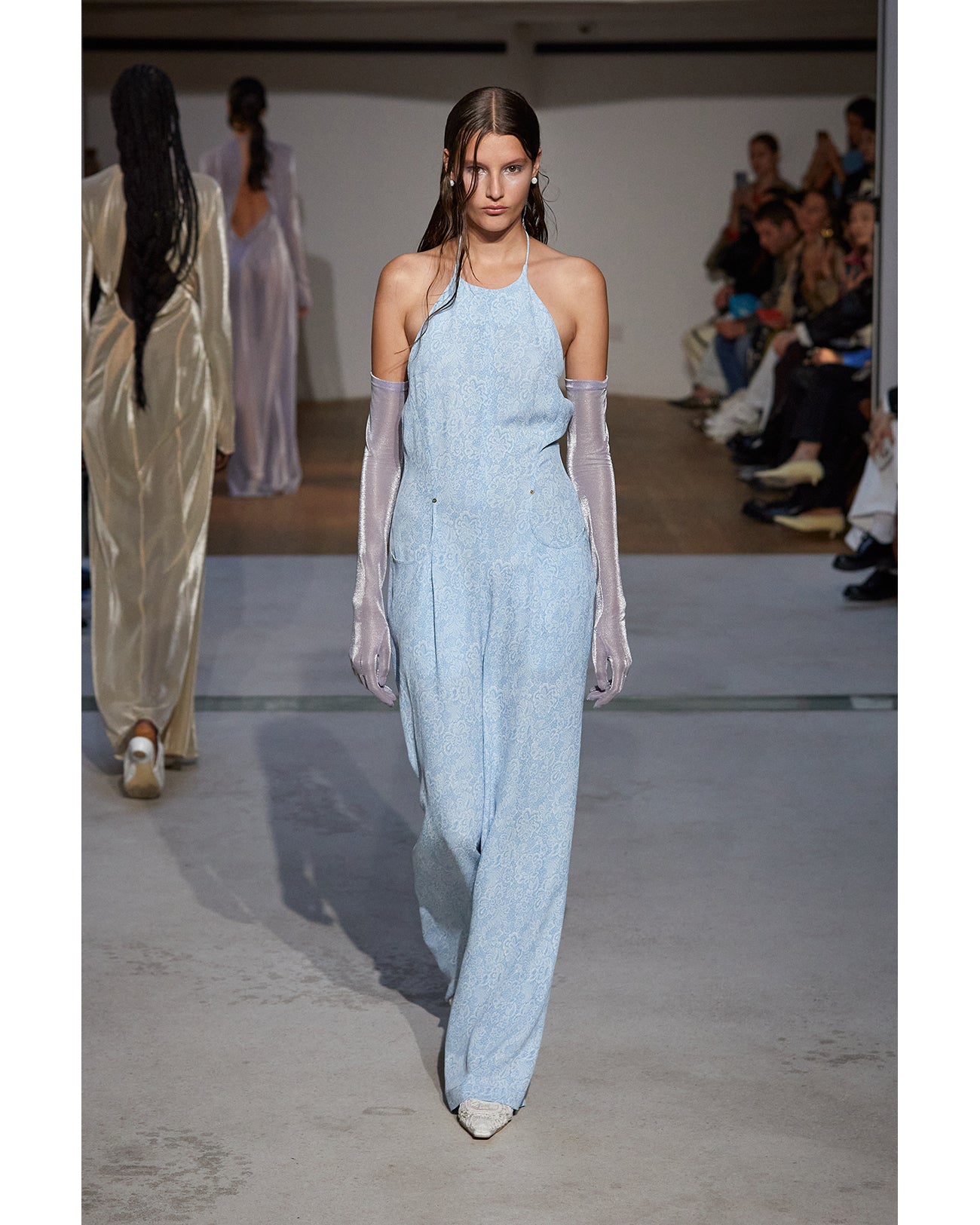In this photograph, a young, tall, and thin Caucasian model, appearing to be around 20 years old, is captured striding down a runway with a composed and serious expression. Her long brown hair flows freely, with some strands cascading over the right side of her face. She dons a light blue halter-neck jumpsuit made of sheer fabric, featuring light white embroidery and displaying her bare shoulders. Enhancing her elegant look, she wears long, silver luminous gloves that extend above her elbows. Complementing her ensemble, she adorns white earrings and white heels. 

To the left of her, another model walks in the opposite direction, dressed in a shimmering gold long dress and silver shoes, with her long brown hair styled in a ponytail. Further behind, another model with long black braided hair, who appears to be African-American, wears a beige silk jumper and white shoes. The runway is covered with a light gray carpet over a parquet floor, and in the background, an audience sits along the right side, attentively observing the fashion show. The setting is minimalist, with white walls and a blend of white marble and brown wooden flooring.